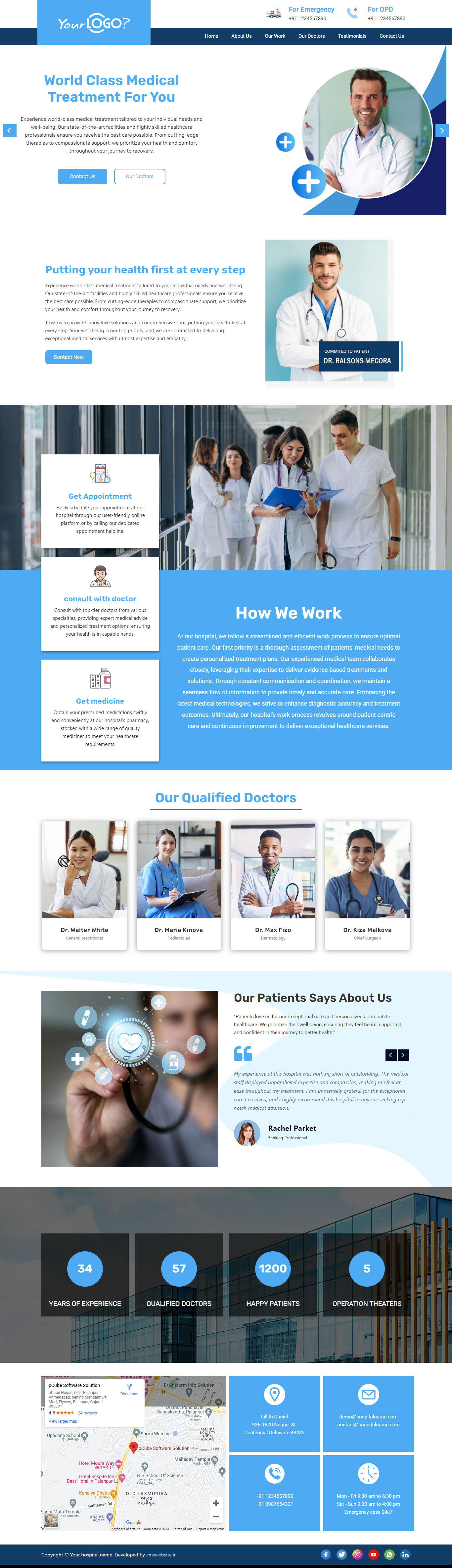This image is a heavily reduced-quality screenshot of a medical website, appearing more like a conceptual mock-up, rendering much of the text difficult to decipher. 

At the top, there's a horizontal black navigation bar stretching across the width of the screen. On the left end, a protruding blue rectangle displays the placeholder text "Your Logo?" in large white letters. The upper right-hand corner features several white menu labels that are too small to read, but above the black bar, "For Emergency" and "For OPD" are slightly visible in blue text. 

Beneath this bar, the main white section of the webpage features multiple paragraphs of text interspersed with images. In bold blue letters, the heading reads "World-Class Medical Treatment for You," followed by two buttons—the one on the left is turquoise, and the one on the right is white, though their labels are illegible. To the right of this text, there's a circular image of a young doctor in his early 30s posed against a white, blue, and dark blue backdrop.

The next section has another blue heading, "Putting Your Health First at Every Step," followed by a paragraph of unreadable text and a rectangular blue bar with white text. Adjacent to this section, there is a square image of another young doctor standing against a blue wall, with a stethoscope draped around his neck. Below his image, a black band displays the name "Dr. Ralson's Macorah."

At the very bottom of the page, a segmented section contains an image of five doctors—three of them women—walking along a corridor or bridge, examining a blue chart. Below this image, the section is blue with white text, which remains indiscernible. To the left, there are three white squares with blue labels and icons, titled "Get Appointment," "Consult with Doctor," and "Get Medicine," each accompanied by an unreadable paragraph. On the right side, in white text on a blue background, it says "How We Work."

Just beneath this, four images of young doctors are displayed horizontally with the heading "Our Qualified Doctors." The subsequent section showcases a doctor holding a stethoscope with a heart icon at its end, accompanied by the text "Our Patient Says About Us" and further unreadable text. 

At the bottommost part of the page, a horizontal black bar houses social media icons on the right—identifiable as Facebook, Twitter, a potentially orange icon, possibly YouTube in red, another in green, and a blue one—and white text on the left side.